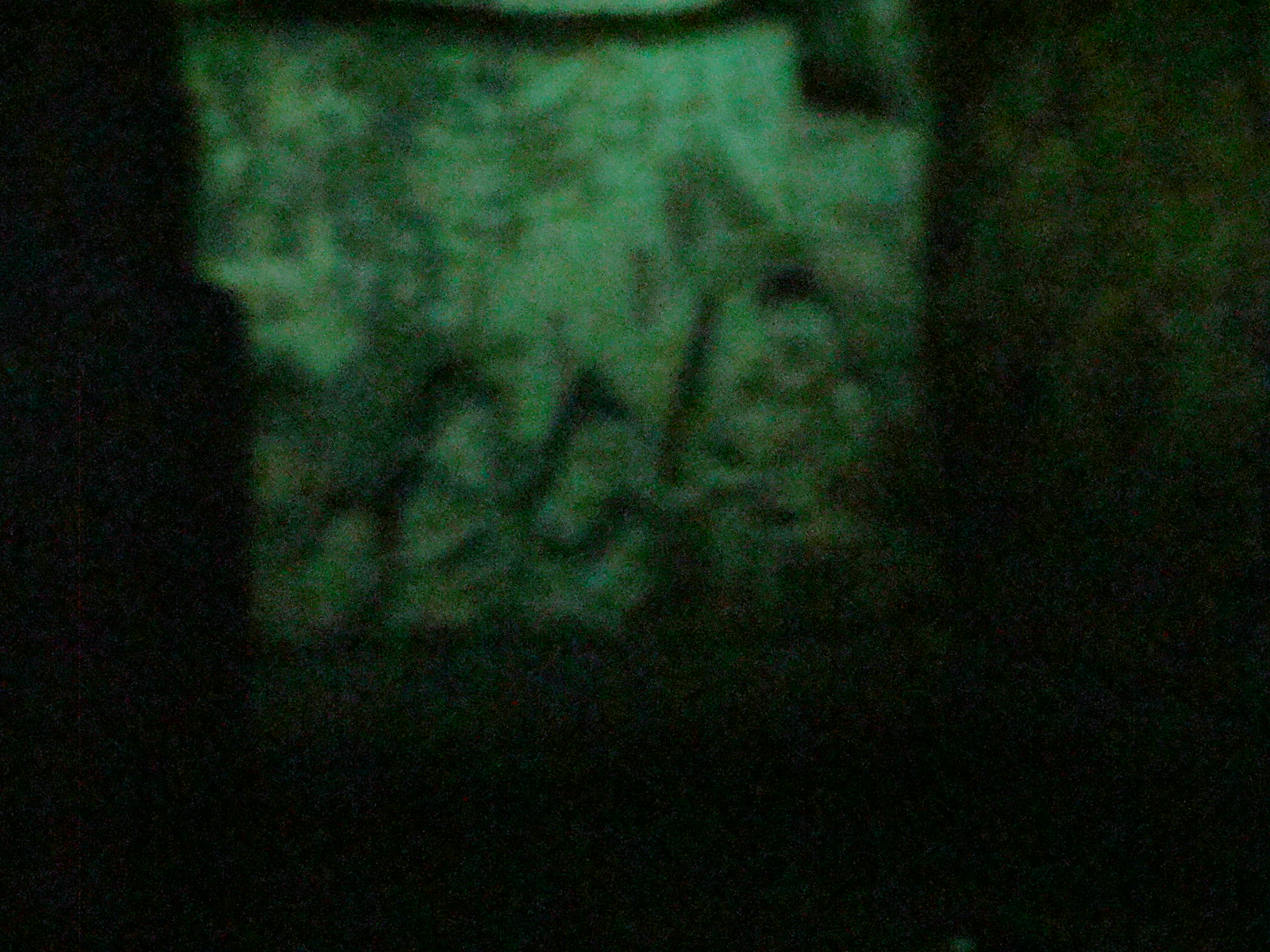The image is a slightly blurry illustration depicted on an object with a whitish background. The top right corner of the image has a small notch taken out of it. The illustration features three or four figures, likely representing historical warriors from centuries ago. These figures have black hair and pale faces, and one of them appears to be carrying a stick with something attached to the end. The object bearing this illustration is situated on a surface, possibly a chair, with part of the chair visible to the right and a bottom cushion seen below.